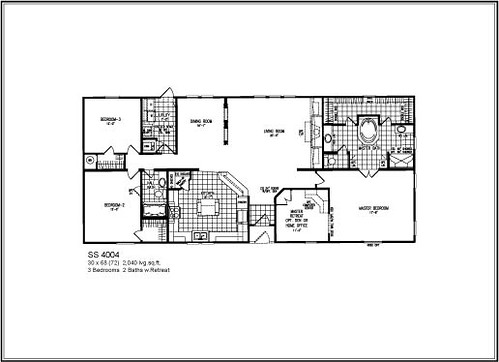This image displays a photocopy of a compact floor plan for a small home or apartment, prominently centered amidst ample white space. The layout comprises three distinct rooms with individual doorways. An open dining area seamlessly connects to a living room, providing a communal space for relaxation and dining.

On one side, a spacious master bedroom is complemented by a large walk-in closet and an expansive master bathroom. Adjacent to the master suite, a kitchen features a cozy breakfast nook. Across from the kitchen, a smaller bathroom offers additional convenience. 

Two smaller bedrooms are situated towards the left, each equipped with modest closets, and a small hallway closet adds extra storage nearby. Almost every room in the floor plan is enhanced with windows, ensuring ample natural light. The foyer serves as the entry point, optimally positioned to lead into the heart of the home.